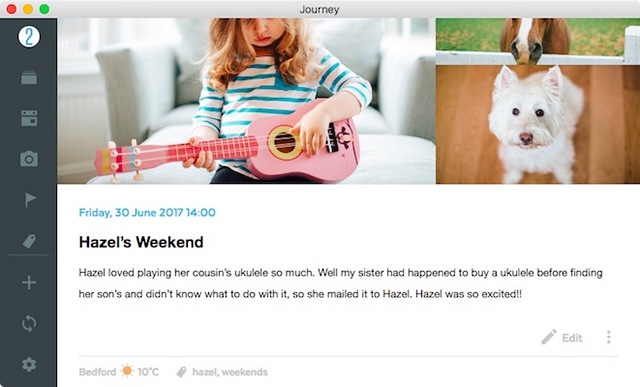This is a screenshot of a Macbook's Journey program interface, displaying a blog-type post. On the left side of the screen, there is a vertical dark grey toolbar with various icons representing settings, refresh, photos, and other functionalities. The main section of the screen features a photograph of a young girl, approximately 4 or 5 years old, enthusiastically playing a pink ukulele. Adjacent to this photo, there is a partially visible image of a horse peering over a white fence, and a small white terrier dog sitting on a wooden floor.

Below these images, the text reads: "Friday 30 June 2017, 14 o'clock, Hazel's weekend. Hazel loved playing her cousin's ukulele so much. Well, my sister had happened to buy a ukulele before finding her son's and didn't know what to do with it so she mailed it to Hazel. Hazel was so excited."

At the bottom right of the screen, there is a weather icon indicating sunny weather in Bedford with a temperature of 10 degrees Celsius. The post is tagged with "Hazel" and "weekends," and there is an option to edit the post.